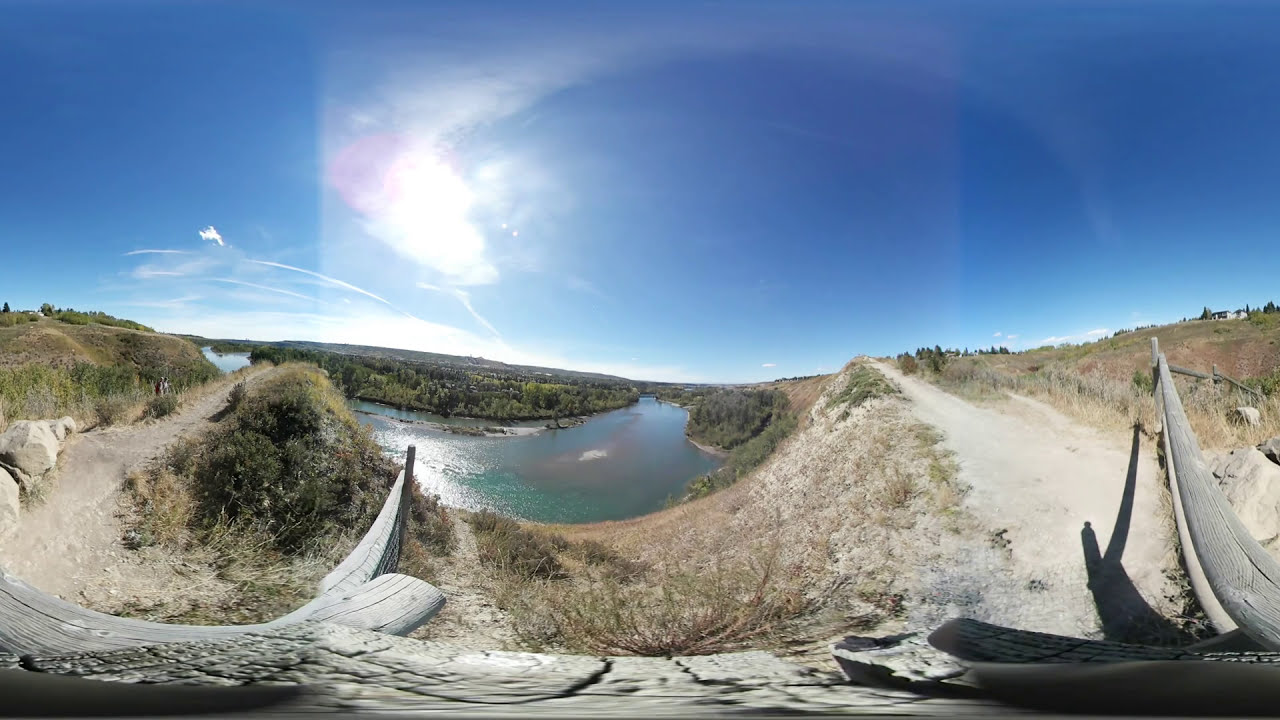This image captures a serene outdoor scene, possibly in a desert or semi-arid region resembling Arizona. Central to the composition is a shallow, aqua-blue river or stream that meanders from the center-left, curves gently to the left, and disappears behind a series of low hills. In the foreground, sandy ground is dotted with shrubs and patches of dark brown grass, adding a textural contrast to the scene. Stretching horizontally across the bottom of the image is a decaying tree stump or log, adding a rustic element to the landscape.

On the right side of the image, the foreground features a dirt or gravel pathway running along a small hill adjacent to the river. Farther in the background, barren land with brown grass extends outward, emphasizing the wild and largely unpopulated nature of the area. The sky above is a vibrant blue with a few clouds, ranging from light, wispy formations to fuller, more substantial clouds.

Additionally, in the upper center-right, there are one or two small buildings on a hill, indicating minimal human presence in this vast, natural space. The scene is bright and sunny, casting a warm light over the clear, dry environment. The landscape curves gently around the blue sky, which deepens in color from robin's egg blue to a richer, darker blue at the top.